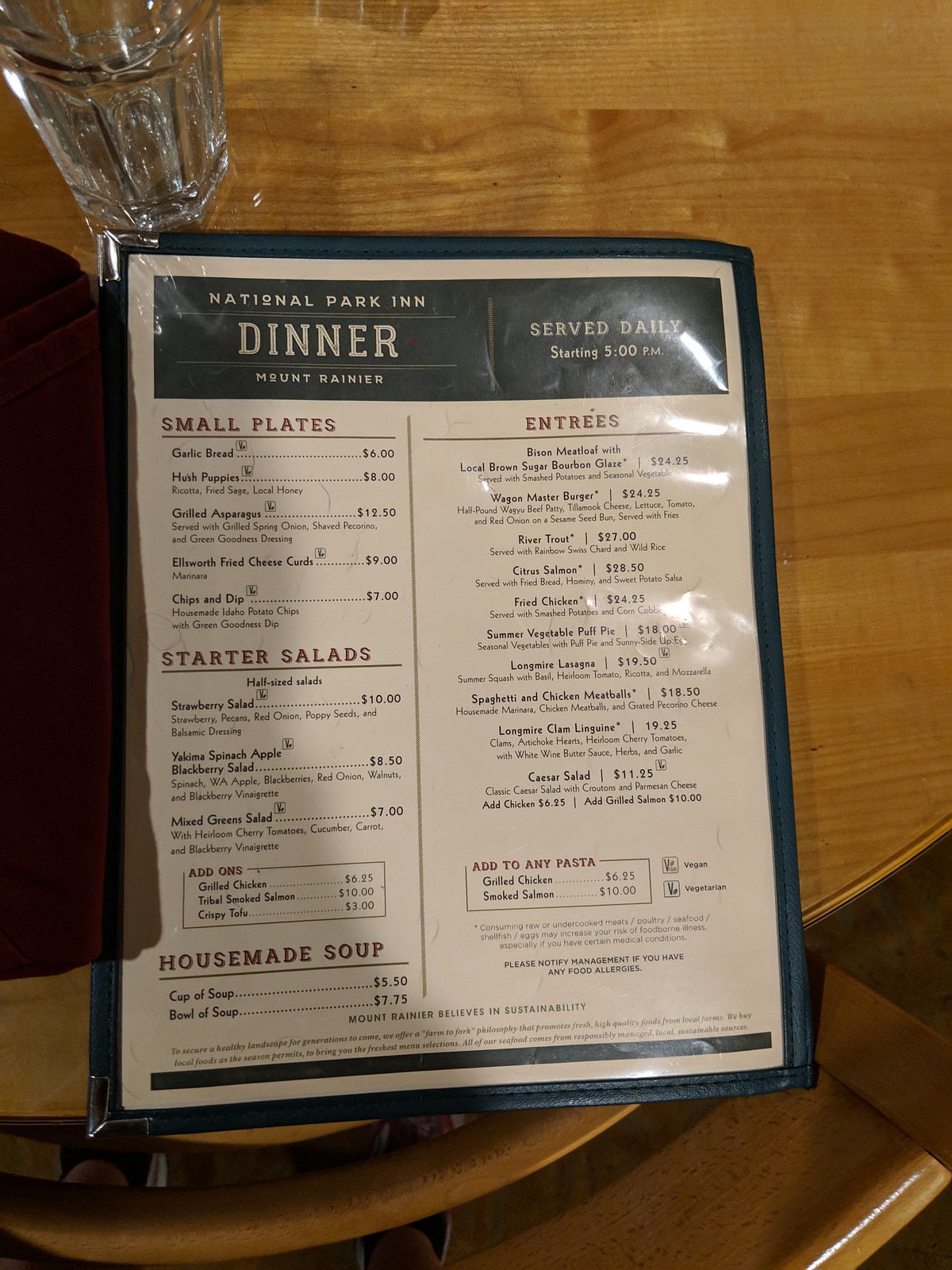This indoor color image captures a top-down view of a wooden dining table with a menu encased in plastic in the center. In the upper left corner, a clear glass filled with water is partially visible. The menu, titled "National Park Inn Diner" with a subtitle "Mount Rainier," features a banner at the top and text indicating that service starts daily at 5 p.m.

The menu is divided into two traditional columns. The left column is categorized as "Small Plates," listing around five or six items, followed by "Starter Salads," and finally "House Made Salads." The right column is dedicated to entrées. Though somewhat blurred, a few discernible items include "Wagon Master Burger," something related to "River Toast," "Cactus," "Fried Chicken," "Lasagna," and "Caesar Salad." The plastic covering the menu reflects light, contributing to some of the blurriness and a light glare on the right side.

A shadow enters the frame from the left edge, just touching the side of the menu, with a slightly rectangular shape suggesting the presence of an object outside the immediate view. In the lower right corner, the back of a wooden chair, matching the color of the table, is also visible, adding to the cozy dining setting.